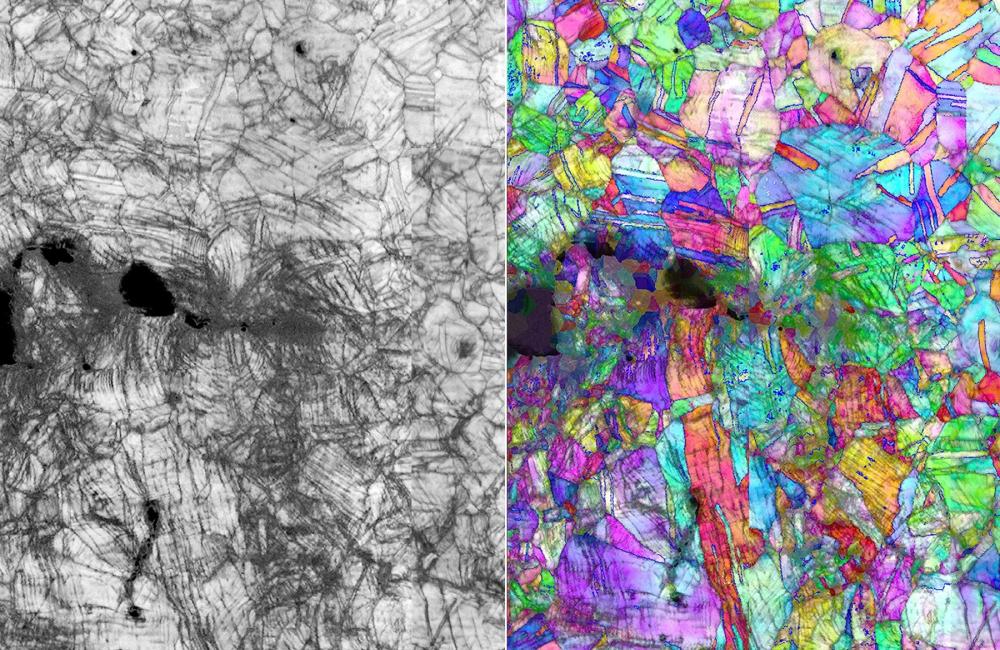This image features two side-by-side, portrait-oriented sections presenting abstract artworks. On the left, there is a black-and-white illustration characterized by a chaotic assemblage of splattered lines, random triangles, irregular shapes, and blotches of black, particularly concentrated on the left side and around the middle. The right section showcases a vibrant counterpart of the left image, resembling a stained glass piece filled with an explosion of colors including gold, yellow, green, blue, pink, purple, red, aqua, and white. Both sections share a similar composition with no discernible pattern, featuring irregularly shaped fragments that fit together. Black splotching is visible on the left side of both sections, reinforcing their connection. The right section amplifies the dynamic energy of the left with its vivid hues, offering a striking contrast to the monochromatic scheme of its companion.